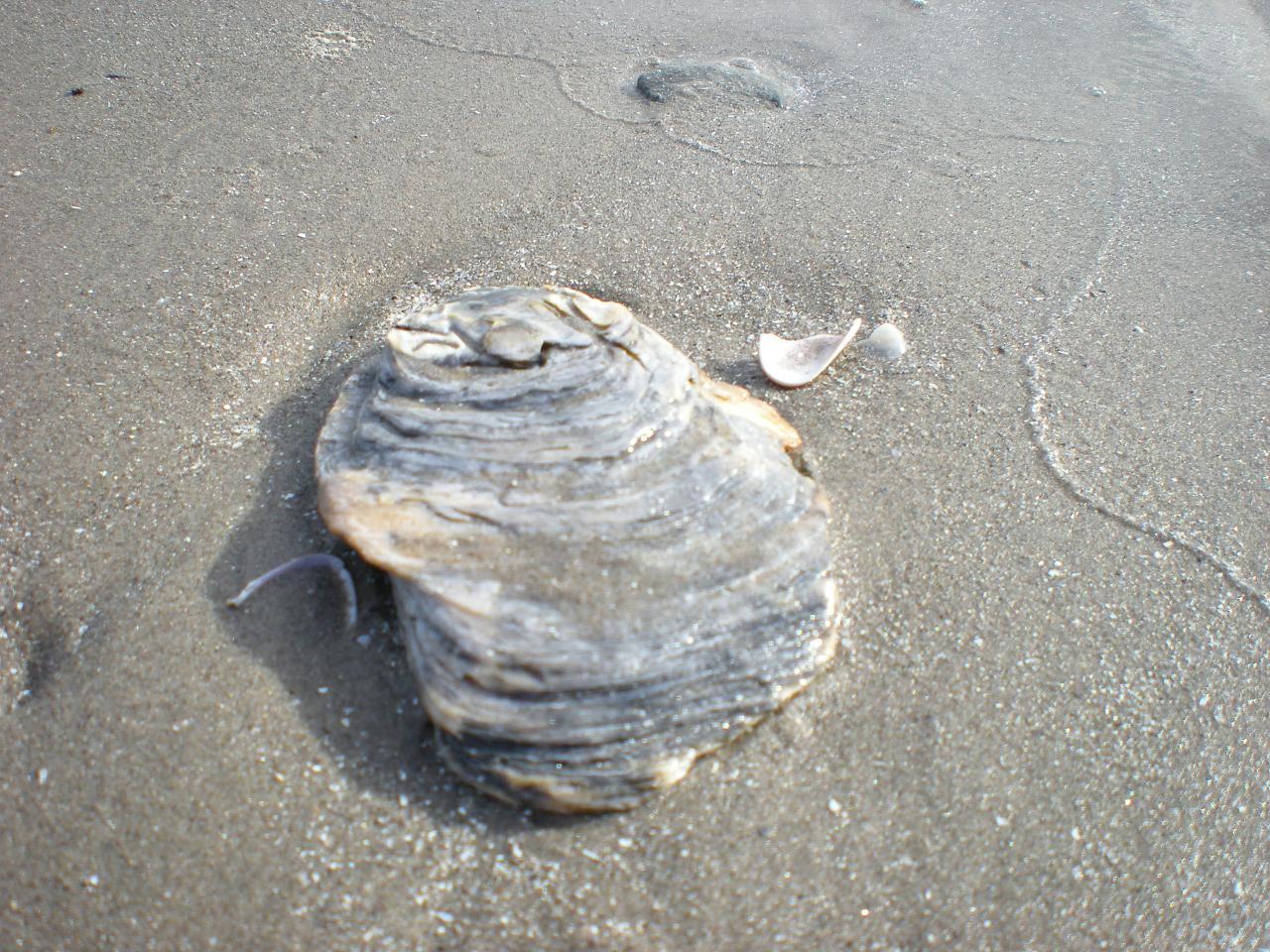The photograph depicts a beach scene dominated by a large, upside-down shell, resembling a soap dish, situated in wet, grayish sand. The shell, prominently located in the center of the image, showcases a blend of dark gray, silver, and black hues with distinctive ring-like folds. Surrounding the shell, particularly to its upper right, are smaller, broken white shell fragments. The dull-colored sand, speckled with white, stretches across most of the background, capturing subtle lines and ripples indicative of recent wave activity. In the upper right-hand corner, a thin sliver of water hints at the shoreline's proximity and the incoming tide.